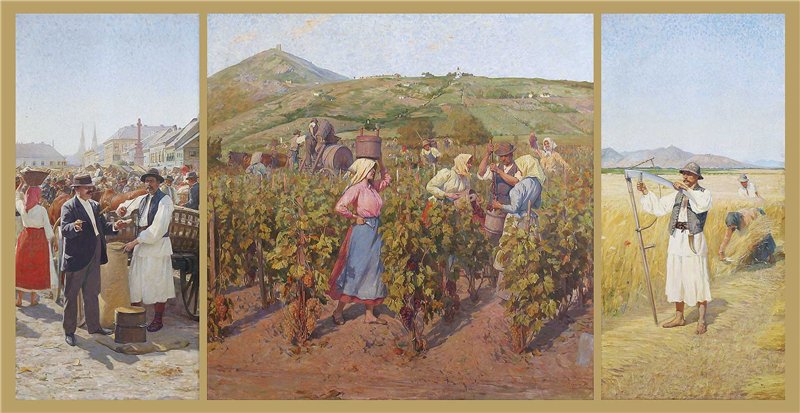This is a detailed painting consisting of three panels enclosed in gold frames, each panel portraying a different scene under a shared blue sky with a city skyline in the background. 

The left panel depicts a bustling marketplace with two men conversing, suggesting a transaction, amidst an array of people. One man, dressed in a suit and hat, is accompanied by a horse-drawn cart, reinforcing the market setting. The scene transitions seamlessly into the middle panel.

The central panel features a verdant vineyard set against rolling green hills and a distant mountain. Workers, including both men and women, are diligently harvesting grapes. The women have their hair tied up with cloth hair ties, and they utilize wooden buckets for collecting the grapes, evoking a sense of communal labor and agricultural activity.

The right panel showcases a light-colored wheat field where workers are engaged in cutting wheat. A man dressed in white with a gray hat is prominently placing or inspecting a scythe. Additional workers can be seen in the background, contributing to the harvest under the clear blue sky.

Overall, this triptych beautifully captures scenes of everyday life, commerce, and agriculture in an old-fashioned setting.